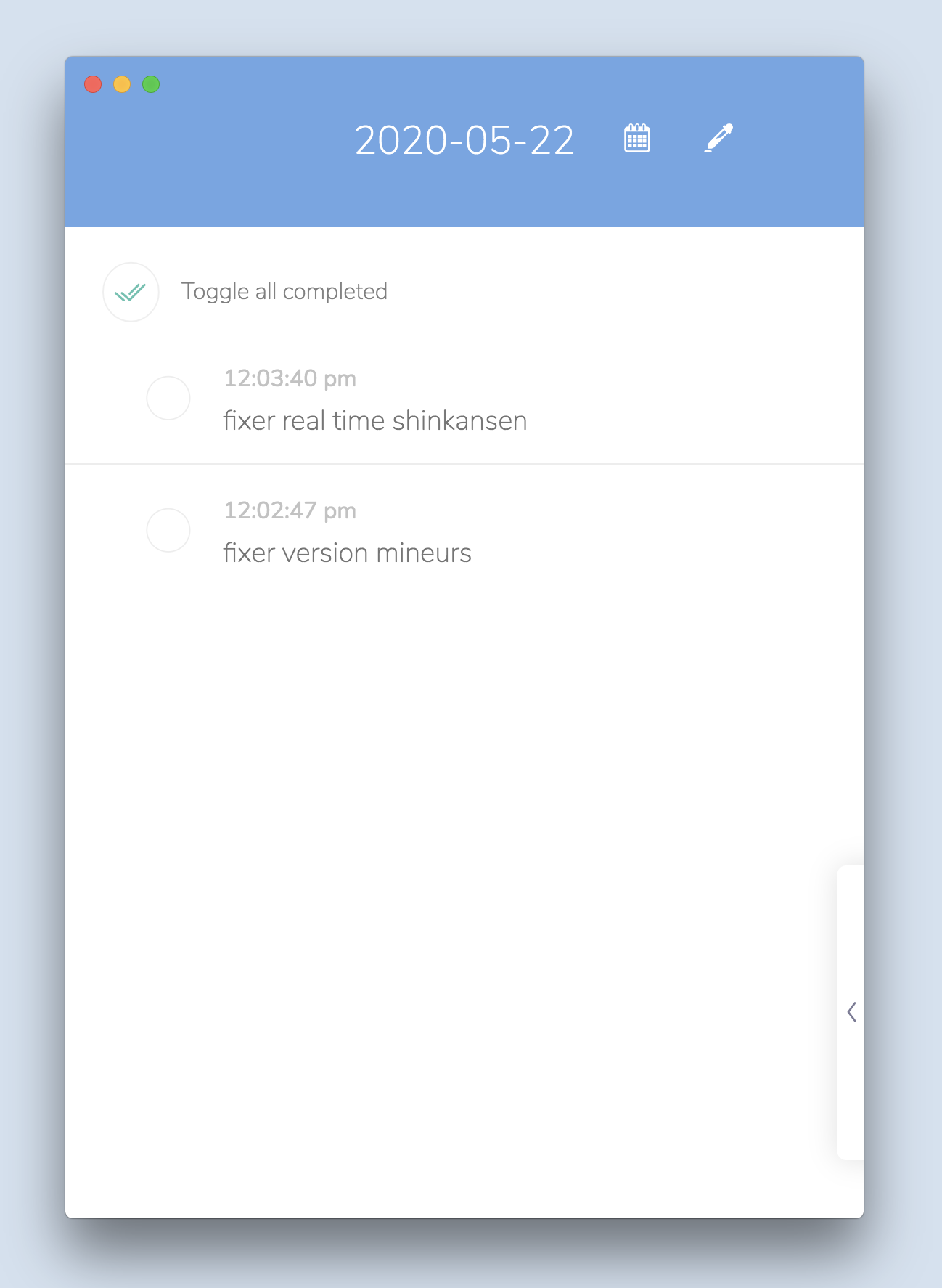This is a detailed screenshot from a mobile device, likely an Android tablet, displaying a reminder or calendar application. The overall background of the screenshot is a serene light blue color. The specific application interface is centrally positioned on the screen, presenting as a wide vertical rectangle.

The upper portion of the screenshot is dominated by a light blue section, featuring three small circles in the upper left corner in red, yellow, and green, commonly representing the close, minimize, and maximize controls of the app interface.

Centrally within this blue area, the date "2020-05-22" is prominently featured, indicating May 22, 2020. Accompanying the date are two small icons: a calendar symbol and a pen symbol, likely signifying calendar events and editing options.

Below this section, the app interface transitions to a white background. At the top of this area is a green checkbox adjacent to a black text line that reads "Toggle all completed," which likely serves as a control to manage task completions.

Further down, the interface bears two distinct reminders. Each reminder entry is separated by a thin horizontal line. The first entry, timestamped at 12:03:40 PM in light grey text, reads "Fixture Realtime Shinkasten" in bold black text. The second entry, slightly lower and timestamped at 12:02:47 PM, reads "Fixture Version Minears," also in bold black text.

Each reminder entry is accompanied by an empty circle, which implies options for user interactions such as selecting or marking the reminders.